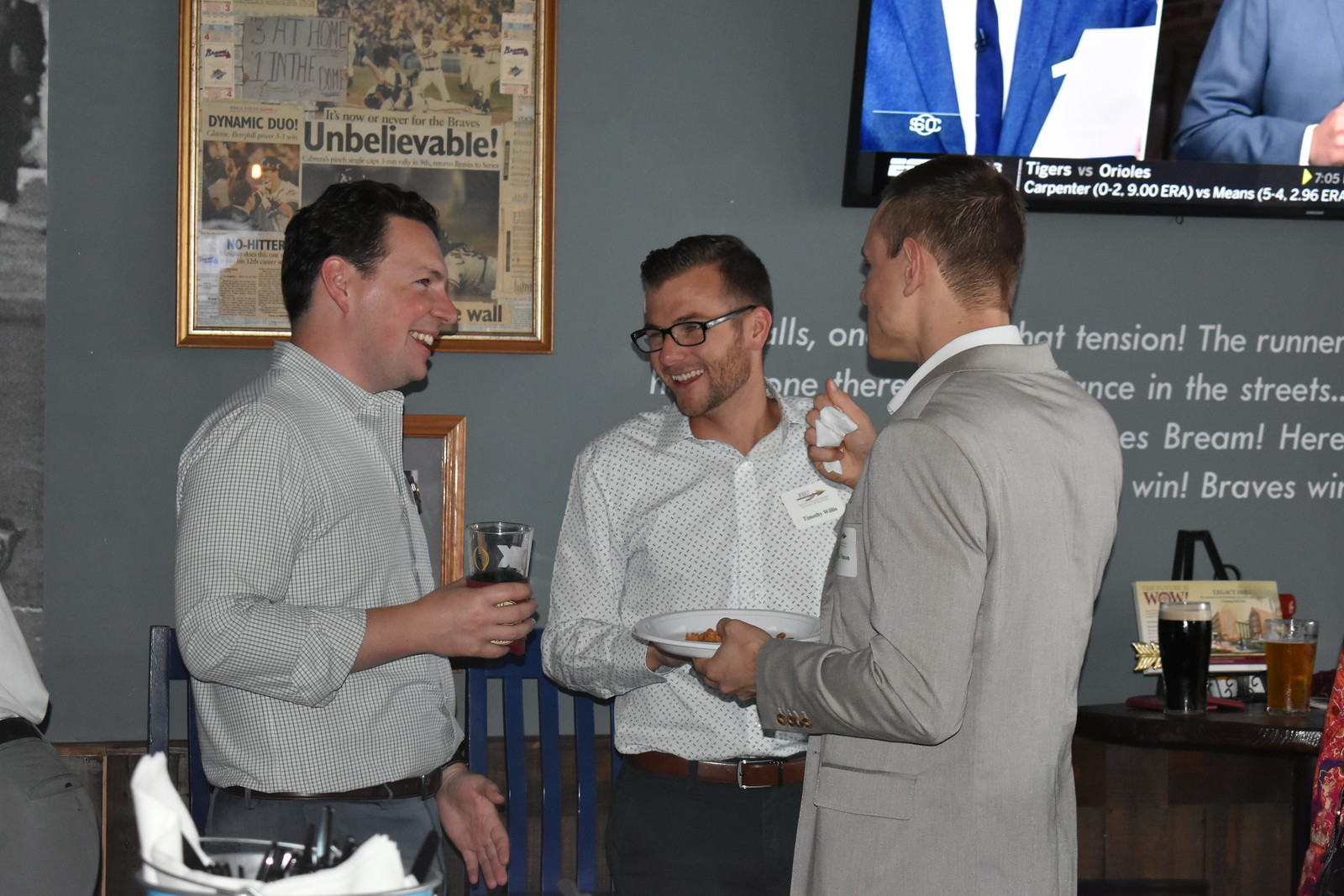The photograph captures three young men, dressed in business casual attire, engaging in a lively conversation at what appears to be a meet and greet event set in a bar environment. All three men are adorned with name tags and have short hair. The man on the left, with short dark hair, smiles as he holds a beer in his right hand and wears a gray and white checkered shirt. The man in the center, sporting a scraggly beard and black-framed glasses, wears a white and black polka-dotted shirt, dark blue pants, and a brown belt. He too is smiling and appears to be the focal point, looking at the third man. The third man is seen from behind, wearing a gray sports coat over a white shirt, with sandy blonde or light brown hair. He is holding a paper plate and a napkin.

The background of the image reveals a typical bar setting with tables partially visible, especially in the bottom right corner, and glasses filled with amber liquid. To the top right, a television screen broadcasts Sports Center. On the top left hangs a framed newspaper article, adding an authentic touch to the bar ambiance. The three men, standing and laughing in a small circle, give off an aura of camaraderie and enjoyment.